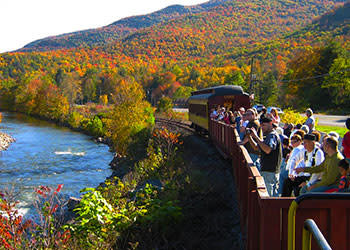In this vibrant and scenic image, a bright sunny day illuminates a picturesque mountain landscape covered in lush greenery and vibrant fall foliage. A trolley car, seemingly designed for tourist excursions, has come to a stop on a bridge, allowing its passengers to disembark and explore the scenic lookout point. The foreground features a colorful array of flowers and dense vegetation, leading down to a serene blue lake or pond. The tourists, armed with cameras, eagerly capture the breathtaking views of the water and surrounding forested mountains, which seamlessly rise behind the scene. The trolley itself is an open-air design, allowing passengers an unobstructed view as they stretch their legs and enjoy the spectacular natural beauty, with the bright sun casting a clear, white hue in the sky above.